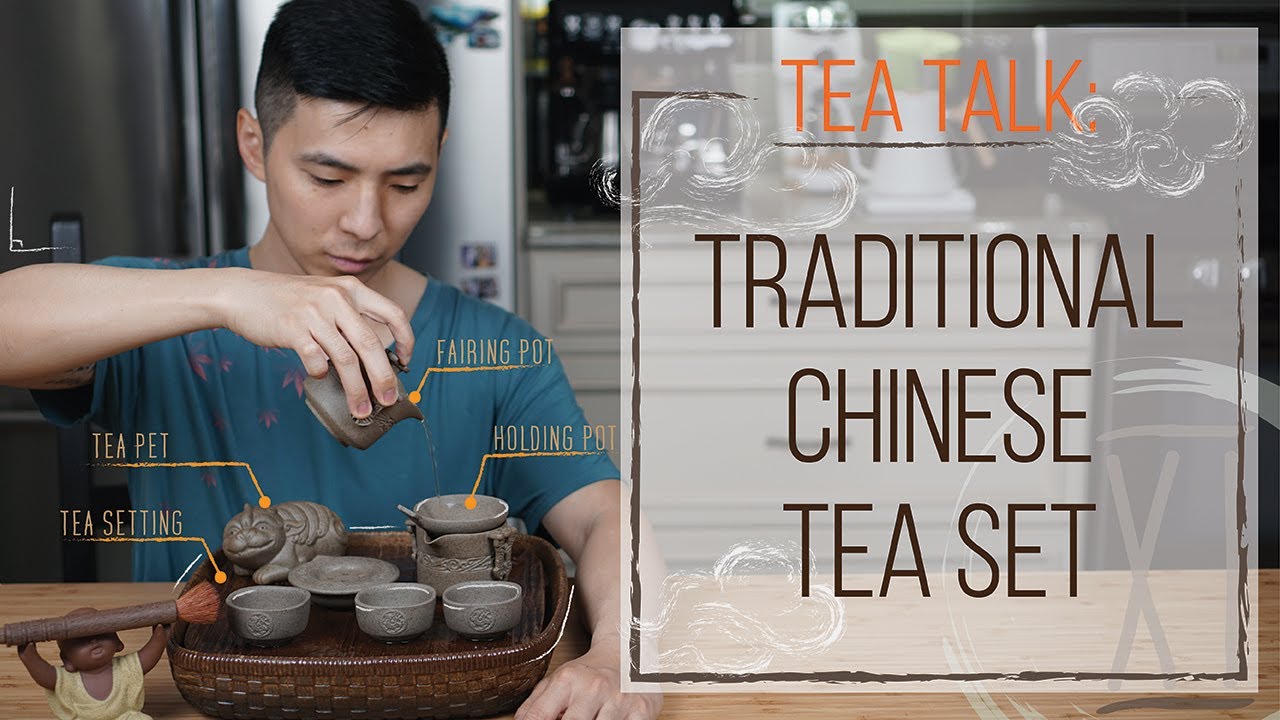This image resembles a promotional material or brochure, featuring an Asian man preparing tea using a traditional Chinese tea set. On the right side of the photograph, a white, transparent frame overlays the background, displaying the words "T-talk" in orange text, and below that, "Traditional Chinese Tea Set" in larger black letters. This frame appears see-through, offering a view of the room behind it. 

On the left side, the scene highlights a young man dressed in a blue T-shirt, seated at a wooden table. In front of him, a brown wicker basket holds various components of a traditional Chinese tea set, crafted from gray ceramic. The set includes a small teapot, a larger holding pot, three teacups, and a figurine that resembles a Cheshire Cat. The man is captured in the process of pouring tea from a small teapot into the larger holding pot. Additionally, there is a peculiar brown baby doll also situated on the table, gripping an oversized brush over its head. The overall setting suggests an intricate and traditional tea ceremony.